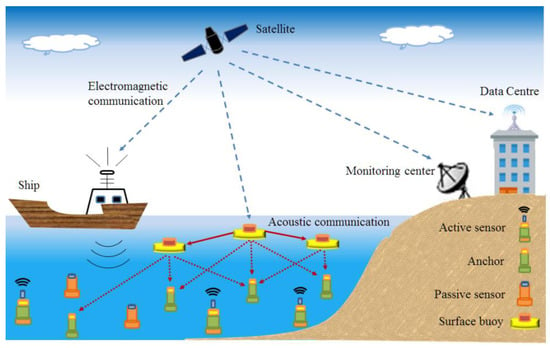The infographic is a detailed, color-illustrated diagram depicting a maritime communication system. At the top of the image, against a gradient sky transitioning from dark blue to white, a satellite labeled "Satellite" emits four dotted blue lines representing electromagnetic communication. One of these lines targets a ship on the left side of the image, another reaches a "Monitoring Center," and the last one connects to a "Data Center" on land to the right.

The midsection of the infographic features a brown ship labeled "Ship," equipped with radar emitting lines and sonar waves penetrating the water below, indicating acoustic communication. The water, shaded in light blue, contains various underwater sensors depicted as green and orange objects resembling traffic cones, identified in the legend as active sensors, anchors, and passive sensors. These sensors are connected via arrows to three surface buoys, yellow with red tops, depicted floating on the water's surface. 

On land, characterized by light brown coloration akin to a sandbar, the "Data Center" building sits alongside a "Monitoring Center" equipped with a satellite dish. The infographic's key explains the function of all elements, highlighting the integrated system where surface buoys communicate with underwater sensors and the ship, relaying information back to land and the satellite. The entire scene, set against a backdrop of two clouds, cohesively illustrates how both electromagnetic and acoustic communications are employed for monitoring maritime environments.